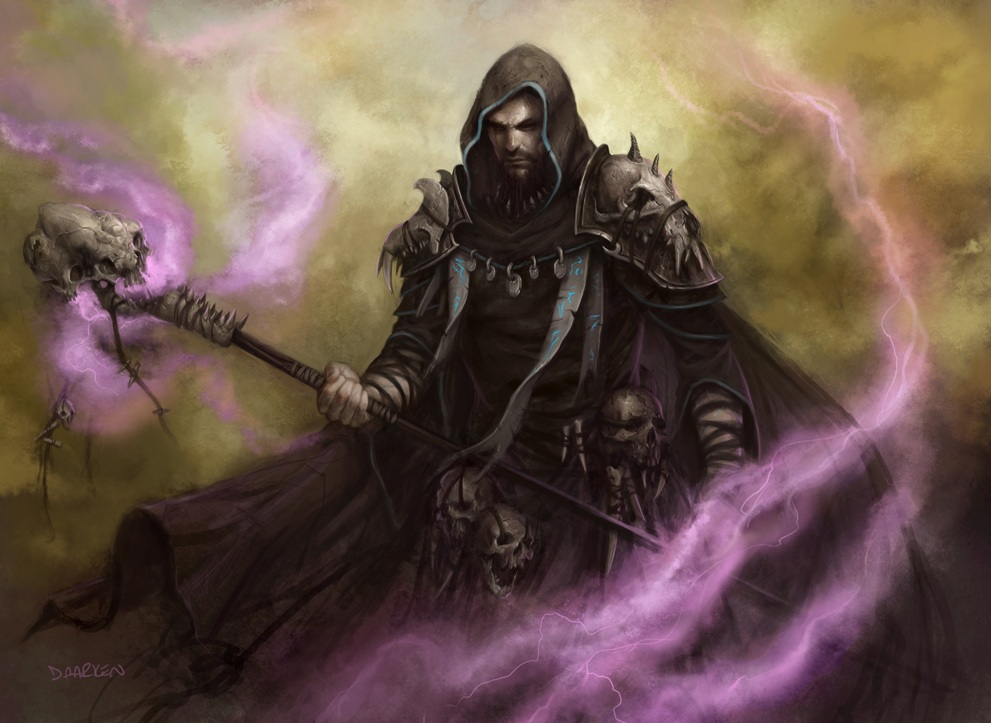The image is a meticulously detailed fantasy artwork depicting a surreal scene with a central mysterious figure. The background comprises a billowy smoke of beige, tans, and brownish-yellow hues, interspersed with white and pink mottled patterns and fluffy lines. Dominating the foreground is a man adorned in a black, hooded cloak edged with thin teal. His shoulders are clad in spiked metal armor, and dark bronze skulls dangle from his attire, adding to his menacing appearance. A black, billowing cape flows around him, enhancing his enigmatic presence. He wields a staff topped with a skull, from which pink, lightning-esque swirls emanate, enveloping him in an ethereal haze. The artwork exudes an unearthly allure, reminiscent of a fantastical video game or an evocative book cover.